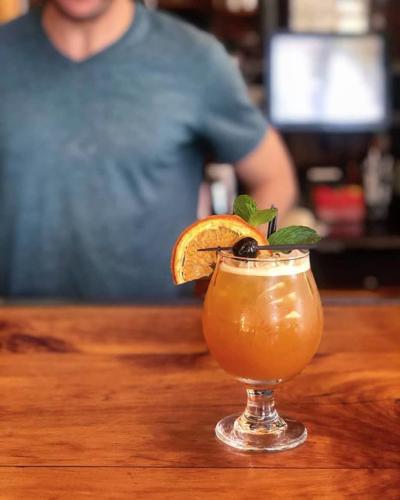The image captures a drink in a sophisticated-looking cocktail glass with a pedestal base and a rounded middle, sitting on a well-finished, stained wood countertop in what appears to be a restaurant or bar setting. The drink itself is amber-colored with a hint of foam at the top. Garnishes include a slice of orange on the edge of the glass and a black olive skewered alongside a cherry and some leaves, possibly herbs, on a toothpick resting across the rim. In the slightly blurred background, there's a young man wearing a blue t-shirt (or possibly a gray t-shirt judging by lighting nuances), likely the bartender who crafted the drink. His shoulder is partially visible, along with his beard, suggesting a casual yet attentive presence. Additional details include a TV set or computer screen and shelves, likely holding bar supplies, adding to the ambiance of a lively, inviting bar. The overall presentation of the drink looks very appealing, making it an ideal promotional image for the establishment.